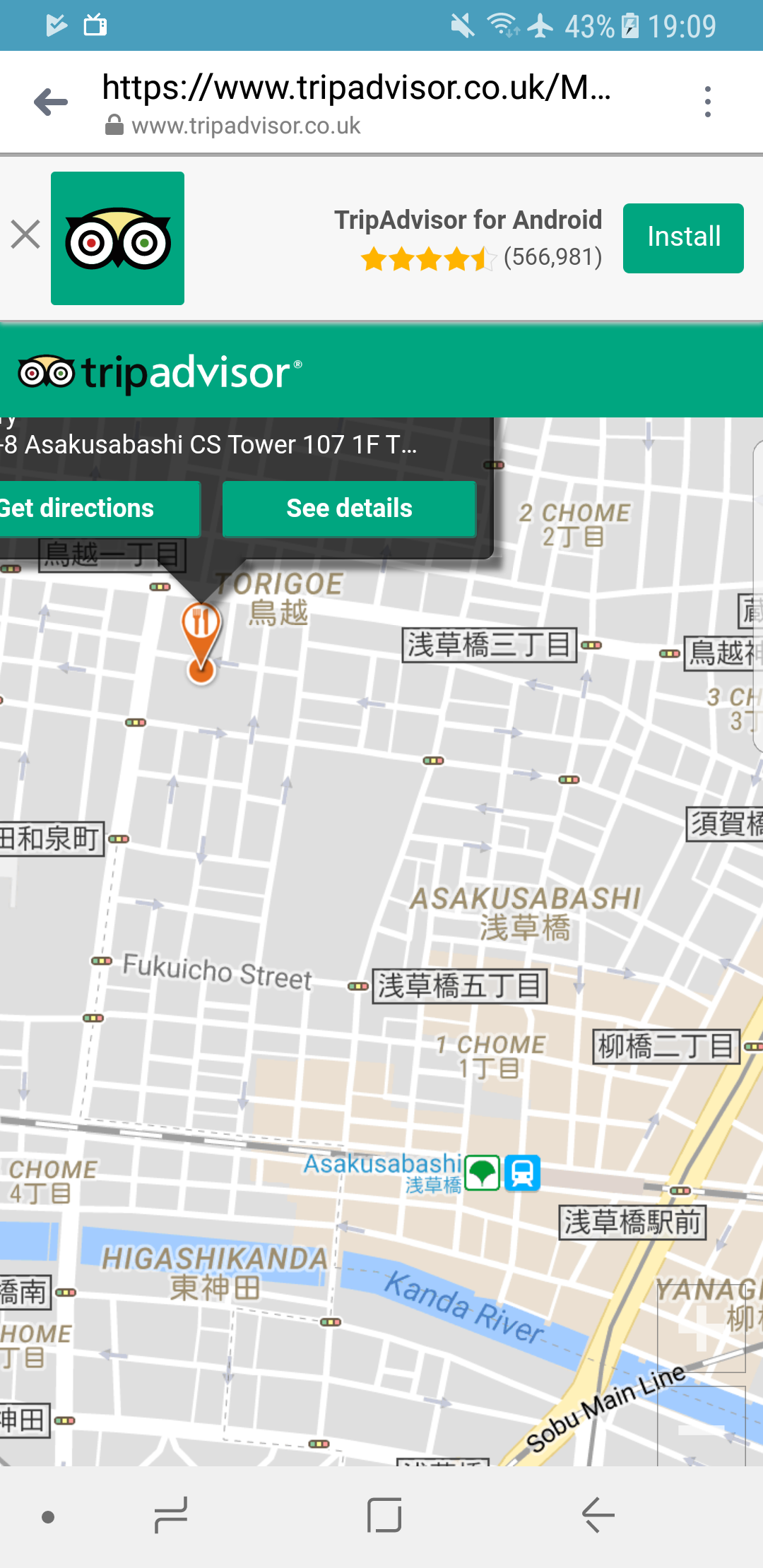The image is a screenshot of a TripAdvisor map displayed on a smartphone. At the very top, the blue phone status bar displays various icons such as a triangle with a checkmark, a TV symbol on the left, and the time, battery level at 43%, airplane mode, silent mode, and Wi-Fi signal on the right.

Below the status bar, there is a search bar containing the TripAdvisor website name, a back arrow icon, and two dots on the right. A small dropdown notification window features an 'X' button on the left, the TripAdvisor logo, "TripAdvisor for Android" text, a rating of 4.5 stars, 566,981 reviews in parentheses, and an install button.

Beneath this notification, the main element of the screenshot is a map, likely of a location in Japan. At the top of the map is a green bar with the TripAdvisor logo and accompanying text. The map itself features various colors including light gray, yellow, and blue, and contains both Japanese and English text marking various locations. A notable feature on the map is a box with an arrow pointing down at a specific food place, offering options to get directions, see more details, and provides the address of the location.

The bottom of the screenshot contains a gray bar featuring a dot, two stacked lines each with an extending line, a box, and a left-facing arrow.